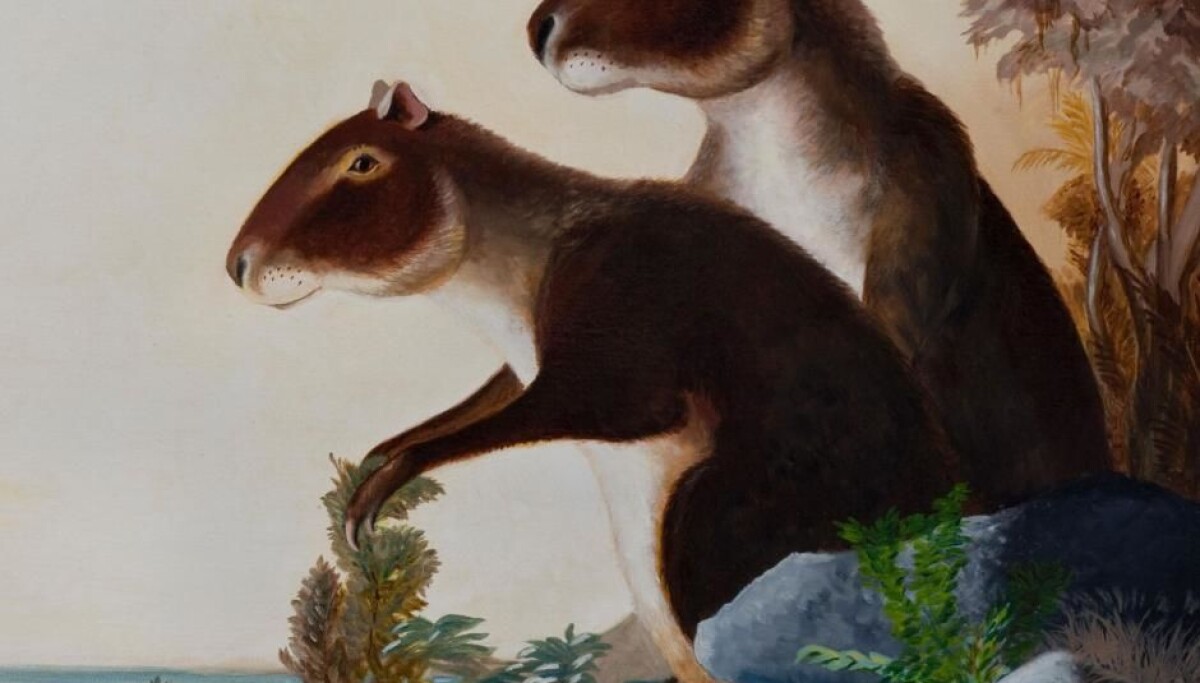The image is a detailed, painted depiction of two large, brown animals with white underbellies that resemble oversized squirrels or possibly groundhogs but could be an extinct rodent species. The animal in the foreground is fully visible, displaying small ears, black eyes, a horse-like jaw, and kangaroo-like limbs with claws. The head of the animal in the background is partially cut off. The scene is set outdoors with a white background behind the animals on the left. On the right, there are brown trees and plants, including gray-yellow branches, a green plant towering over a dark gray boulder, and another gray stone. The detailed illustration captures the texture of the fur and the scale of the animals, which appear larger than the natural elements around them.